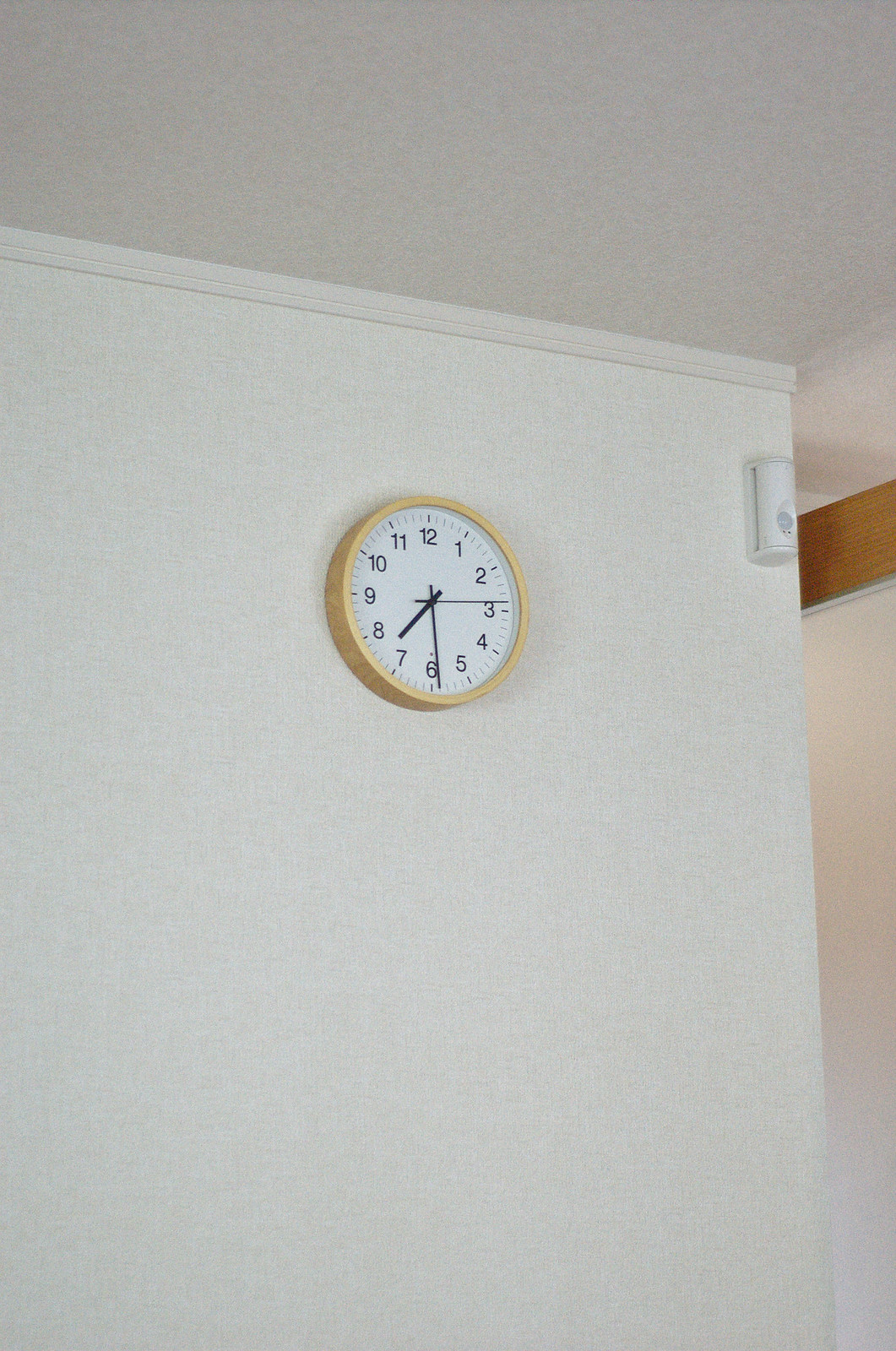Hanging near the corner of a white-walled room, a meticulously detailed clock is mounted high on the wall, approximately a foot and a half below the ceiling. This analog clock, displaying a time near 7:29, features black hour, minute, and second hands against a pristine white background. Surrounding the classic face, which clearly presents each numeral in an upright position, is a plastic frame designed to mimic light wood, blending subtly with the room's aesthetic. Adjacent to the clock is another wired device, symmetrically positioned to the left. Illuminated softly from the right by indirect lighting, the clock and its surroundings create a serene yet precise focal point in the otherwise monochromatic corner.